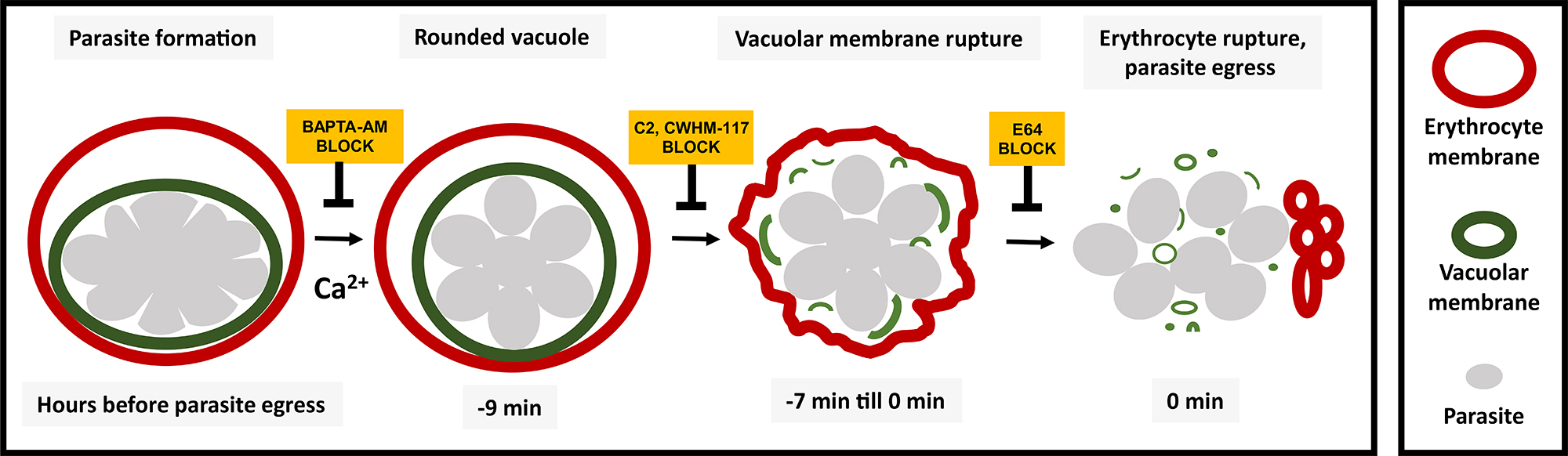This infographic illustrates the process of parasite egress in detailed steps, likely sourced from educational material. The left side features a sequence of images enclosed in a large rectangle with a white background. This sequence is divided into several stages labeled across the top as: "Parasite Formation," "Rounded Vacuole," "Vacuolar Membrane Rupture," "Erythrocyte Rupture," and "Parasite Egress." 

Each stage displays a red circle representing the erythrocyte membrane, a green oval representing the vacuolar membrane, and gray shapes depicting the parasite. Initially, during "Parasite Formation," the parasite is contained within the green vacuole inside the erythrocyte. As time progresses, detailed by labels such as "-9 minutes," "-7 minutes," and "0 minutes," the infographic visually depicts the vacuole and membrane rupturing. During the final stage at "0 minutes," the vacuole ruptures, showing the parasites breaking free into smaller blobs as they egress.

Adjacent to this process on the right side is a vertically oriented rectangle that serves as a key. This key includes a red oval labeled "Erythrocyte Membrane," a green oval labeled "Vacuolar Membrane," and a filled gray oval labeled "Parasite," clarifying the elements depicted in the main sequence.

The infographic is devoid of any human figures and focuses purely on the scientific visualization of this parasitic process, employing a color-coded scheme to enhance clarity and understanding.